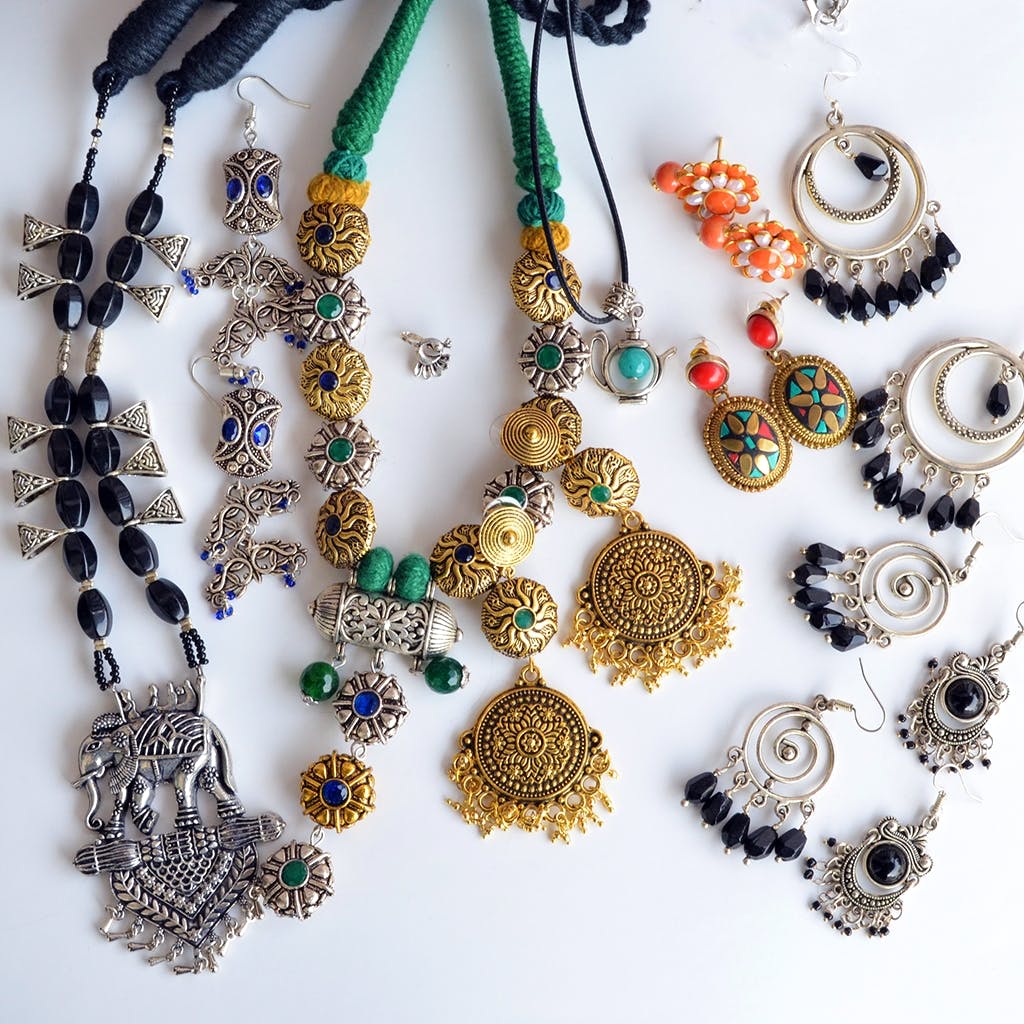This photograph showcases an intricate display of costume jewelry meticulously arranged on a flat white surface, captured from an overhead perspective. On the left side, a black and silver-toned necklace stands out, intricately crafted with black thread and an array of beads in both black and silver. The necklace features a striking silver-tone elephant pendant adorned with ornate henna-style designs, depicting people riding atop the elephant. Directly to the right of this necklace, there is a pair of silver-tone dangling earrings, adorned with tiny blue beads and oval blue gemstones.

Continuing to the right, a second necklace made from green and dark yellow thread draws attention with its disc-shaped beads, alternating between golden and silver tones. Each bead is embellished with green or blue gemstones at the center. Nestled within this necklace lies a small, standalone silver-tone charm, absent of any chain attachment. Next in line is another distinctive piece: a necklace featuring a blue teapot-shaped bead suspended from a black leather cord.

Below the teapot necklace, a pair of statement earrings in gold tones catches the eye. These earrings consist of two large vertical circles, one featuring a jade-colored stone. Spanning from the middle to the far right of the photograph are five additional sets of dangling earrings. Highlights include a gold-tone pair with pearl and orange stones, a silver-tone set resembling hoop earrings with black briolette beads, and another set featuring intertwining silver swirls with dangling black stones. Each set of earrings showcases a unique blend of designs and materials, contributing to the diverse and visually engaging collection presented in the image.